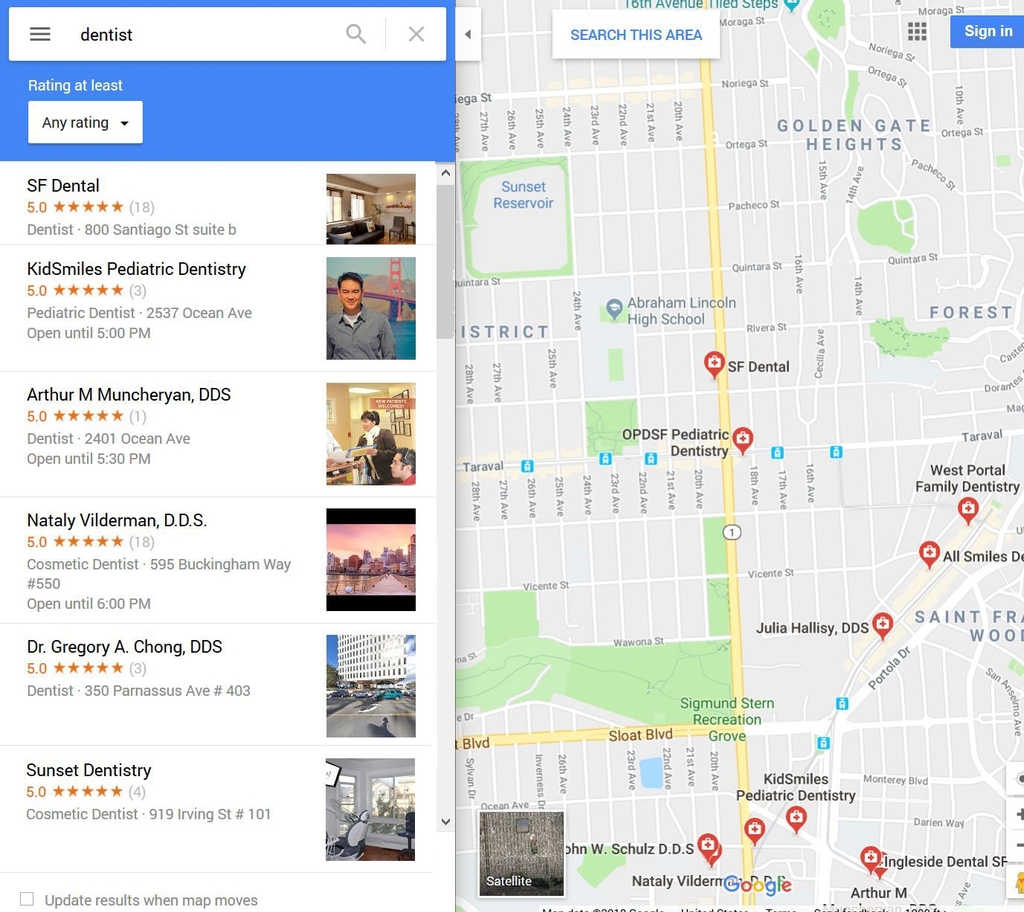The image depicts a screenshot of a Google Maps search interface where an individual has entered the keyword "dentist" into the search bar located at the top left. To the left of this search bar, there is a hamburger menu, and to the right, a magnifying glass and an X icon. Just below the search bar, there is a filter labeled "Rating at least," accompanied by a dropdown box displaying "Any rating."

Below this filter, six dentist locations are listed. The first location is "SF Dental," followed by "Kid Smiles Pediatric Dentistry," "Arthur M. Muncherin, DDS," "Natalie Vilderman, DDS," "Dr. Gregory A. Chong, DDS," and finally "Sunset Dentistry" at the bottom.

On the right side of the image, the Google Maps visual section is displayed, showing a map of the San Francisco area with the label "SF Dental" prominently visible. At the bottom left of the map, there is an option for satellite view, and the bottom middle features the Google logo. Toward the top right, there is a blue sign-in box with the words "Sign in" written in white, and at the top center, a prompt that says "Search this area."